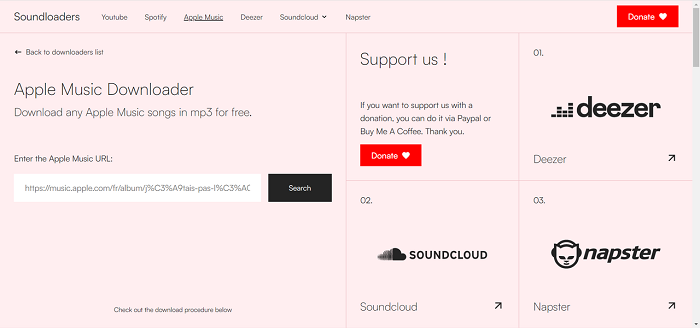A cropped screenshot from a web page, focusing solely on the page content without any browser information, has a light pink background and a grey window scrollbar on the right. At the top left corner, there is a logo for "Soundloaders" in grey text. Below it, a navigational menu lists various music streaming platforms, including YouTube, Spotify, Apple Music, Deezer, SoundCloud, and Napster.

On the left-hand side of the image, there is a box labeled "Apple Music Downloader," accompanied by the instruction "Download any Apple Music songs in MP3 for free." Below this, there is a text entry box containing a long HTTPS web link, labeled "Enter the Apple Music URL," and a black search button adjacent to it.

On the right-hand side, there are four distinct squares, each providing different pieces of information: the first box encourages users to support the site with donations, the second offers a link to Deezer, the third connects to SoundCloud, and the fourth directs to Napster. Each square pertains to a different music streaming service.